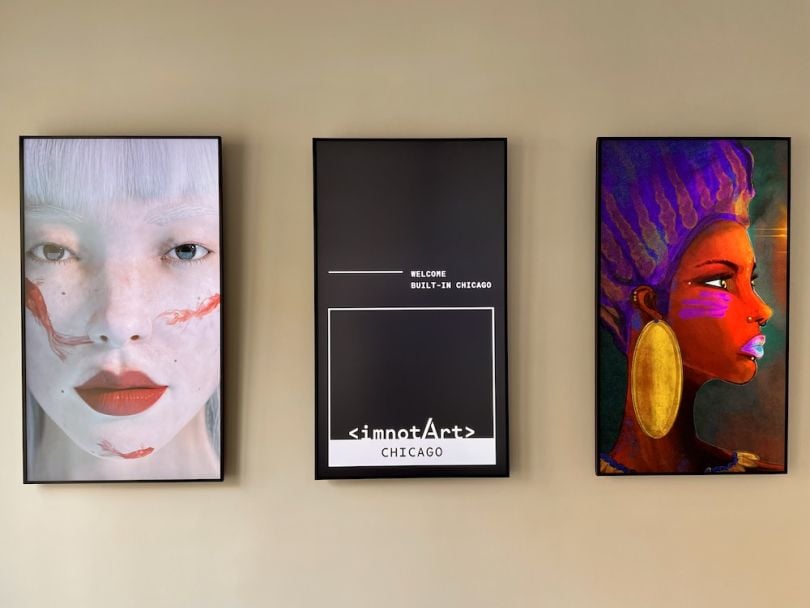A beige gallery wall displays three images, each encased in a thin black frame. The leftmost image appears to be either an ultra-realistic drawing or a photograph of a young woman with pale skin, white bangs, and stark white eyebrows. Her striking appearance is accentuated by large, vivid red lips and a distinct red streak, possibly paint or blood, that extends from her right cheek, across the bottom of her nose, and reappears on her left cheek and chin. The central image is a black sign with the words "Welcome Built-in Chicago" in white text, accompanied by two additional elements: a white square with the phrase "I am not art," where only the 'A' is capitalized, and a white rectangle at the bottom stating "Chicago" in black text. The rightmost image depicts a dark-skinned woman in profile, adorned in traditional African attire. She wears a vibrant purple and yellow headwrap, large gold oval earrings, and has boldly colored makeup with purple on her cheek and pink and blue on her lips.